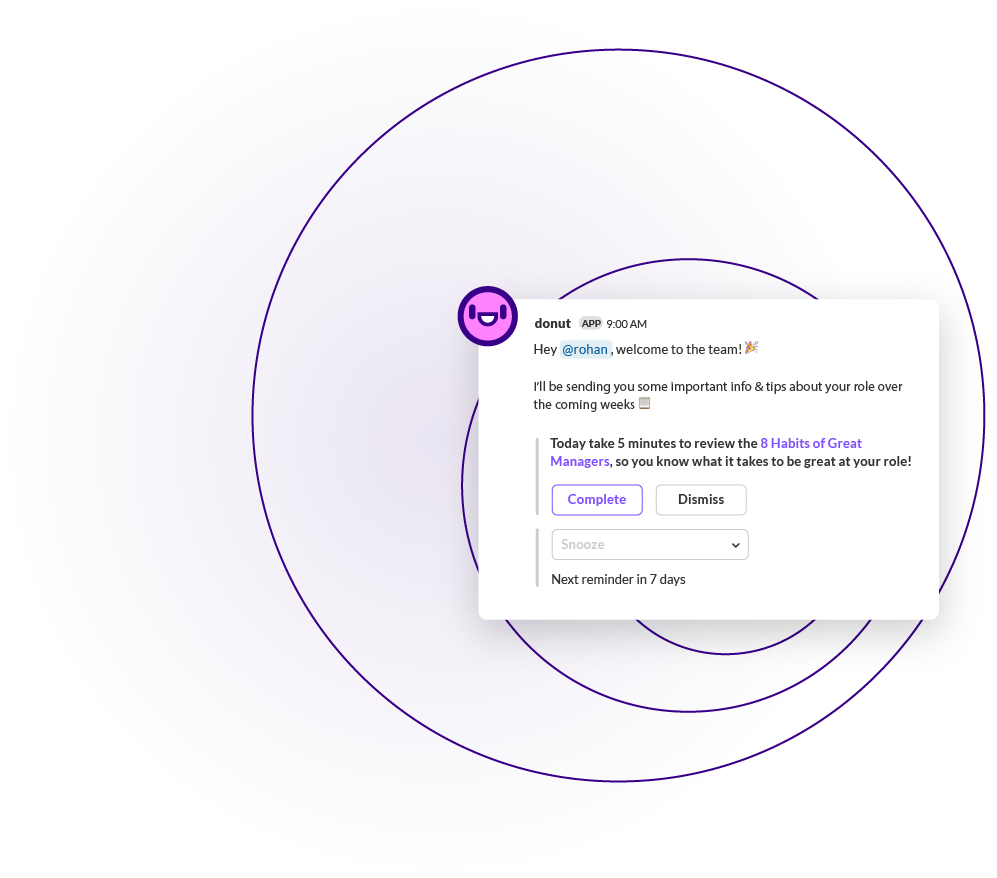The image features a light purplish-white background with a curvy, circular funnel-like pattern. In the center, a white square box obscures most of the background. Inside the box, at the top left corner, there is a purple circle with a smiley face. The text next to the circle reads:

"Donut, 9am
Hey Rohan, welcome to the team!

I'll be sending you some important info and tips about your role over the coming weeks.

Today, take five minutes to review the eight habits of great managers so you know what it takes to be great at your role."

Below this text, there are two buttons: a light purple button labeled "Complete" on the left, and a black button labeled "Dismiss" on the right. Under these buttons, there is another button labeled "Snooze." At the bottom of the box, it states: 

"Next reminder is in seven days."